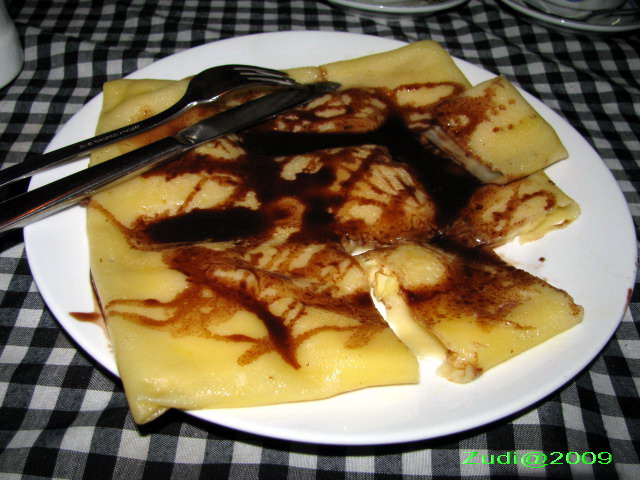The image is a full-color, indoor, staged photograph centered around a white plate of ravioli drizzled with balsamic sauce, creating a contrast with the yellow pasta. The silver fork and knife rest across the top left corner of the plate. The background features a black and white checkered tablecloth that extends to the top of the image, with additional white saucers and a cup or bowl visible in the background. A green text stamp reading "Zudi at 2009" is present at the bottom of the image. The composition showcases the meticulously arranged elements, emphasizing the culinary centerpiece against a stylish backdrop.